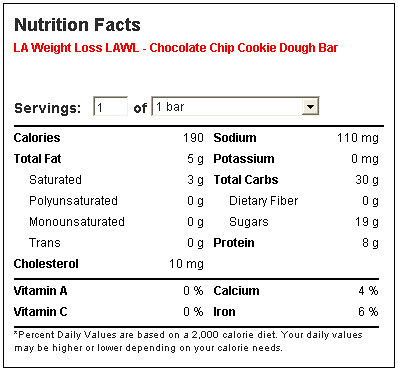The image depicts a square food label with a thin black outline. At the top, in bold black letters, it states "Nutrition Facts." Directly below, in red type, it reads "LA Weight Loss" followed by "LAWL Chocolate Chip Cookie Dough Bar." The label indicates that the serving size is one bar. Key nutritional information is presented: 190 Calories, 5g Total Fat (3g Saturated Fat, 0g Polyunsaturated Fat, 0g Monounsaturated Fat, 0g Trans Fat), 10mg Cholesterol, 110mg Sodium, 0mg Potassium, 30g Total Carbohydrates (0g Dietary Fiber, 19g Sugars), and 8g Protein. Additionally, it includes micronutrient values: 0% Vitamin A, 0% Vitamin C, 4% Calcium, and 6% Iron. It notes that Percent Daily Values are based on a 2000 calorie diet and advises that individual values may vary based on specific calorie needs.